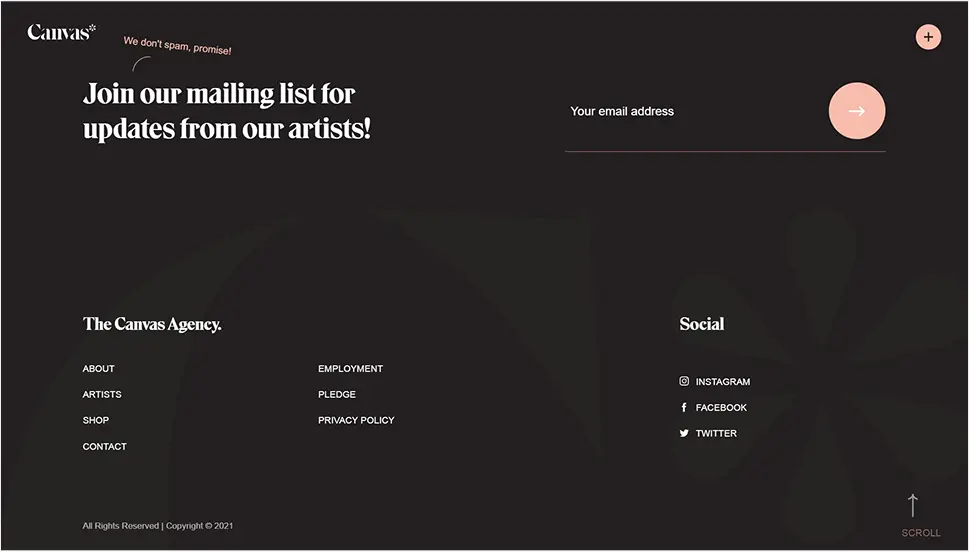This image features a screenshot of the Canvas website set against a black background, prominently displaying a large, watermark-like C and asterisk logo. In the upper left corner, the website name "Canvas" is mentioned alongside the message "Join our mailing list for updates from our artists," followed by a promise in smaller pink text that reads, "We don't spam, promise." To the right, an email entry field is provided with a light orange arrow pointing to the right. The upper right corner of the page features a pink circular button with a plus sign.

A navigation menu in white text includes links to "About," "Artists," "Shop," "Contact," "Employment," "Pledge," and "Privacy Policy." At the bottom of the page, social media icons and links for Instagram, Facebook, and Twitter are listed under the heading "Social," along with an arrow labeled "scroll" in the bottom right corner. The footer contains the statement "All rights reserved, copyright 2021."